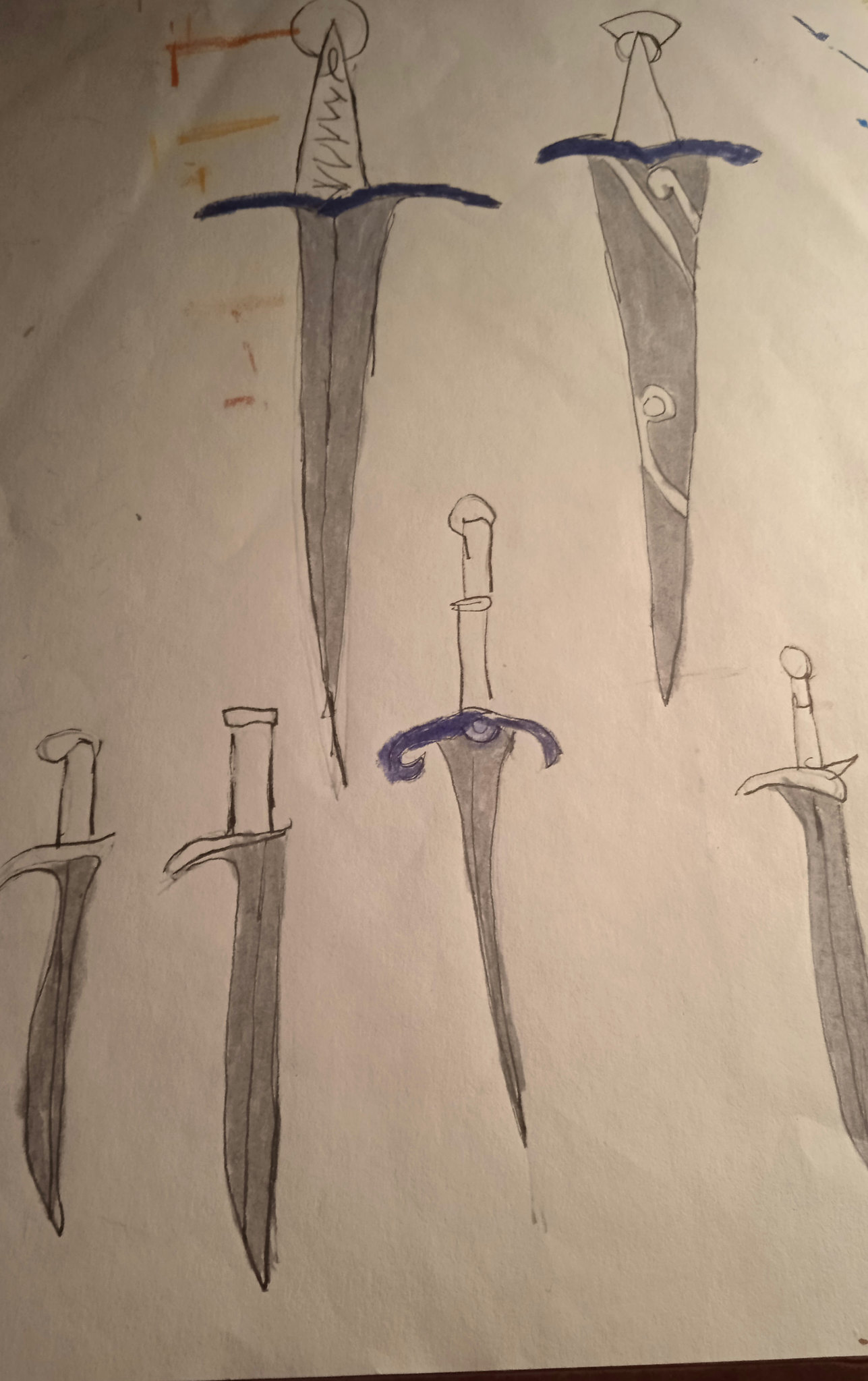This is a photo of a homemade drawing, likely done by a child, on a white sheet of paper featuring six swords. All swords are sketched with a pencil and colored partially with markers. The blades of the swords are uniformly silver, possibly colored with a silver marker. Several elements appear in deep purplish-blue, providing accent to the designs. 

The first sword has a round top handle, transitioning into a triangular section with squiggly lines, followed by a slightly V-shaped blue hilt, and a lined silver blade. The second sword features a capped top, a circle intersected by a triangle, a curved blue line, and a silver blade with a central line and two white swirls. The third sword, located on the bottom left, includes lines extending from the side of the top to the bottom, a partly curved black line, and a slightly curved silver blade.

To the right, the fourth sword has a small rectangle atop a larger one forming the handle, capped off with a curved section converging on the right, accentuated by a central line on the silver blade. The fifth sword is characterized by a cap, followed by a series of rectangles, a curved blue section with a partial non-blue circle, and a silver blade. The last sword on the far right has a circular top, a rectangle with a line, and a combination of a curved line and a triangle on the right side, culminating in a silver blade with a central line. Additionally, there are some partially visible colored letters in orange and yellow at the top left of the page, enhancing the drawing.